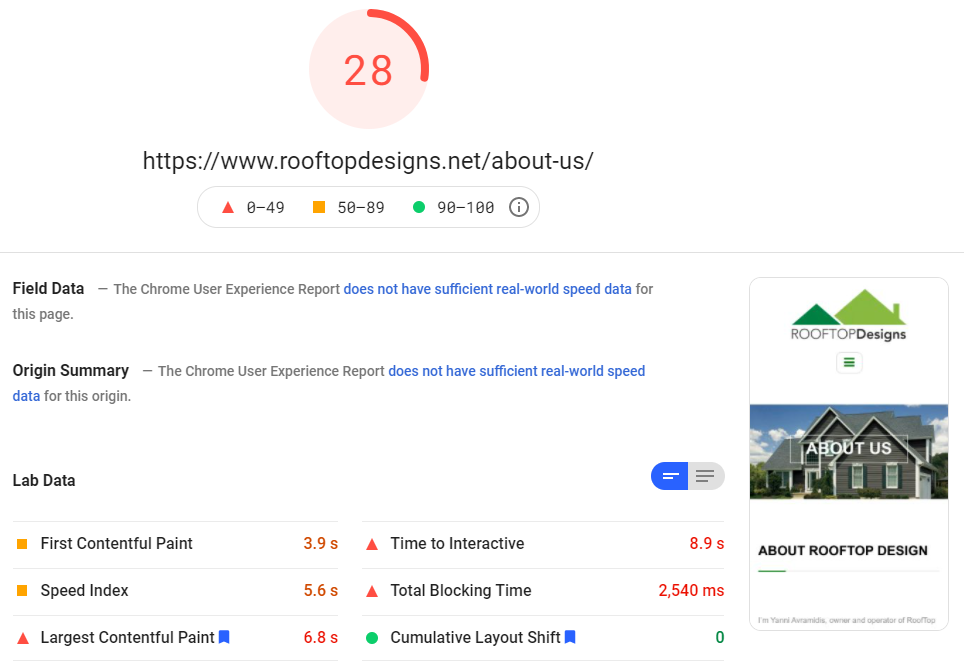The image displays a section of a web page diagnostic tool, most likely related to website performance analytics. At the top-left corner, there is a light red circle with the number "28" inside. This circle seems to be part of a loading indicator, evidenced by a dark red segment partially surrounding it. Below this indicator, the URL "https://www.rooftopdesigns.net" is displayed.

Under the URL, a performance rating legend is shown. It includes a red triangle labeled "0-49," an orange box labeled "50-89," and a green circle labeled "90-100." Adjacent to these, there is an icon of an eye inside a circle. 

Further down, a gray line separates the previous section from the next segment, which focuses on field data. On the left, the text "Field Data" is displayed, followed by a note from the Chrome User Experience Report, highlighted in blue, stating that there is insufficient real-world speed data for the page, presented in black text.

Below this, an "Origin Summary" section reiterates that the Chrome User Experience Report, again highlighted in blue, lacks sufficient real-world speed data, presented in black text for the origin. Finally, further down, the "Lab Data" section includes a performance metric: an orange square with the text "First Contentful Paint 3.9s."